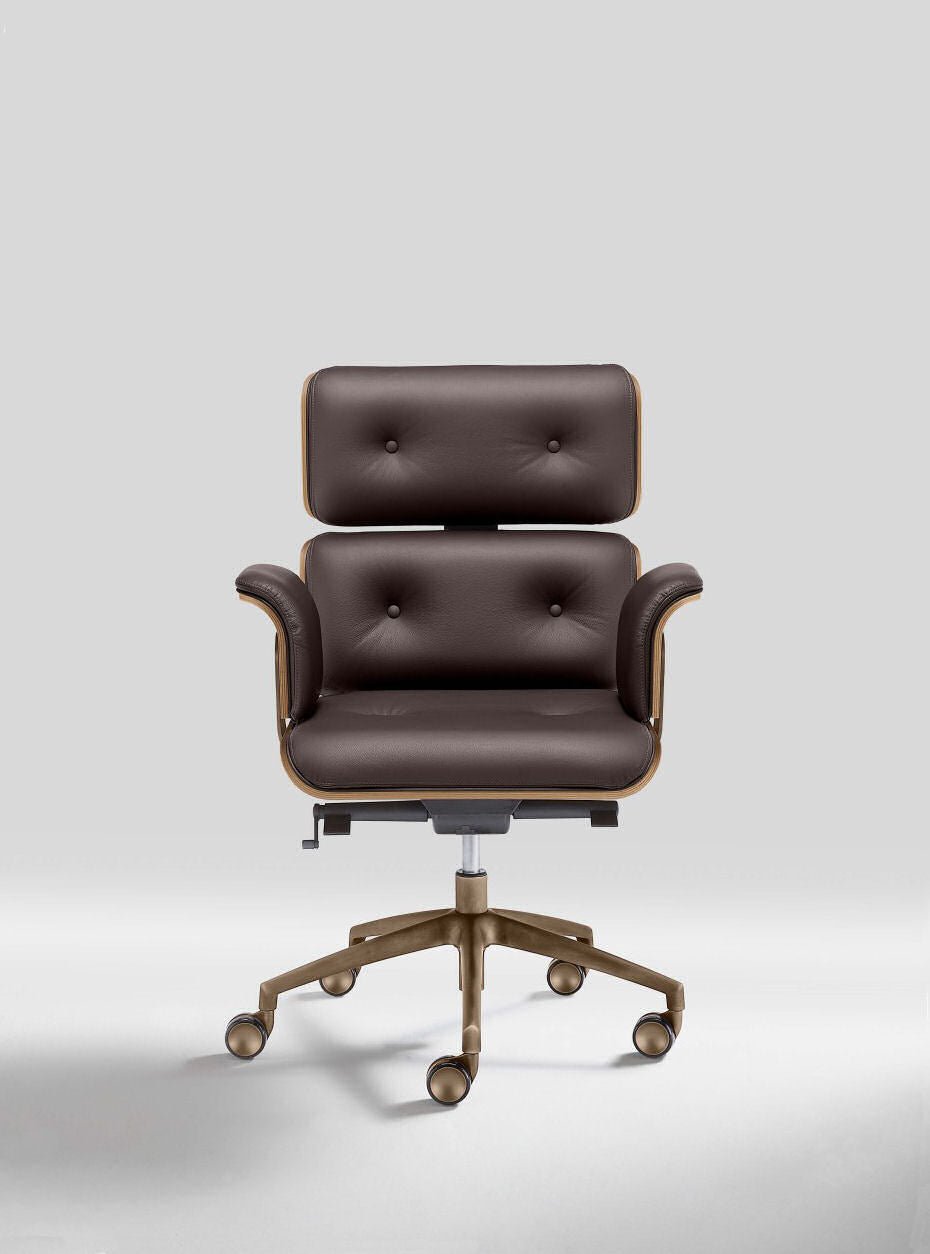This photograph features a detailed product image of a luxurious office chair presented against a plain white background. The chair itself is constructed from dark brown leather and includes generous cushioning for added comfort. Its backrest is composed of two rectangular pillows, a larger one on the bottom and a smaller one on top serving as a headrest. The seat and armrests are also padded with leather, and the armrests curve gracefully up from the sides of the seat.

The chair is supported by a sturdy base with five copper-colored roller wheels, which allow for smooth mobility. Visible underneath the seat is a small toggle switch for height adjustment, connected to a chrome bar. The part where the handle is attached is solid black, providing a striking contrast to the overall design.

Photographed facing directly towards the viewer, the chair’s design details, including its wide, rectangular back and well-padded seat, are clearly visible. The image is shot at a straight-on angle, enhancing the chair's prominence against the clean, white backdrop that features subtle shadowing, giving a slight gray tinge to the floor and wall. This meticulous setup emphasizes the chair’s new, pristine condition, making it stand out as an elegant and functional piece of office furniture.